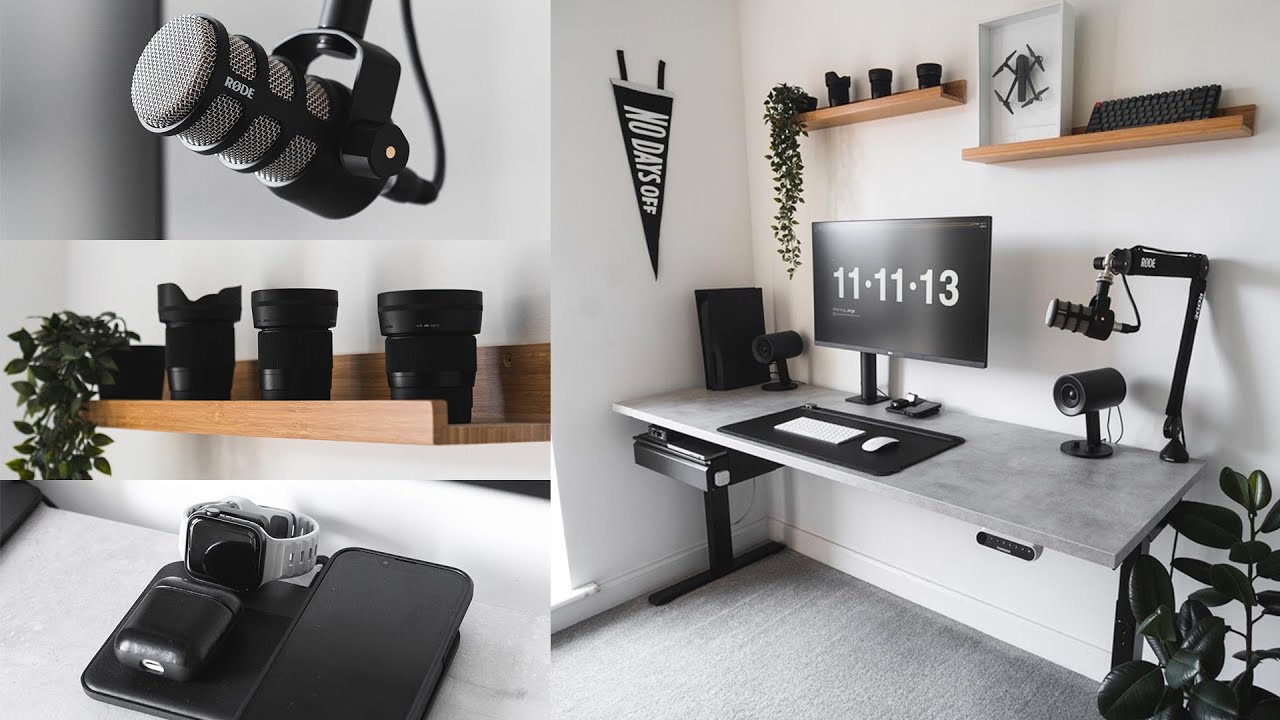The image showcases a meticulously organized home office desk setup, presented in a collage of four photographs. The top left image features a black RODE microphone against a white wall, identifiable by its unique "Ø" symbol. Below it, the second photograph displays a set of four small black planters on a wooden countertop, with only the far-left planter hosting a thriving plant. In the third picture, a smartphone is seen resting on a charger, accompanied by a smartwatch resembling a Fitbit, all placed on a white surface.

The fourth and largest image on the right provides a zoomed-out view of the entire desk setup within a white-walled room. A gray marble countertop hosts a computer monitor with a white keyboard and mouse on a table mat. The RODE microphone is visible alongside a black camera, while a black pennant with "No Days Off" in white letters hangs on the wall. Directly above, there’s a shelf holding three camera lenses and a vase with a plant.

The room features additional details including a black PS5, a drone, and two cameras or lights flanking the monitor, showing the blend of productivity and tech interests of the occupant. The desk, supported by black legs, has certain unidentified equipment stored beneath it. The overall theme of the room is minimalist and clean, dominated by black, white, and gray tones, with occasional touches of green from the plants. The flooring is a shade of gray, further complementing the modern aesthetics of the room.